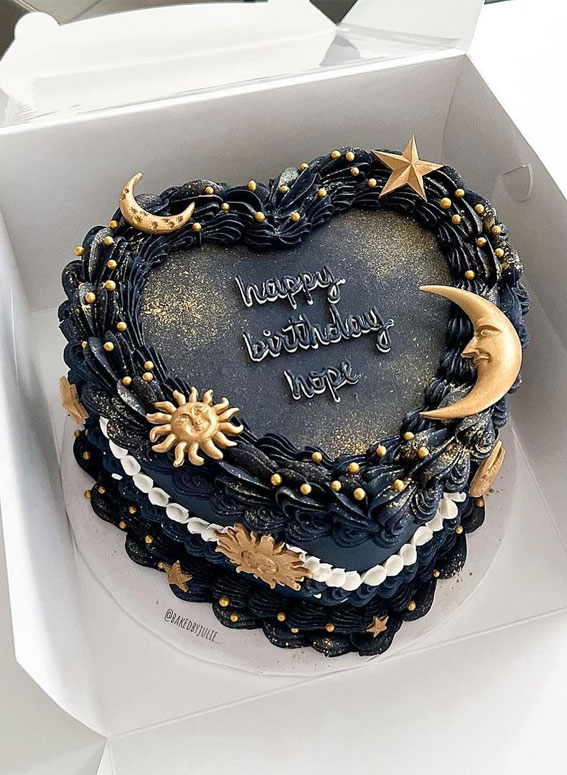Inside a white cardboard box with the lid open sits a heart-shaped birthday cake adorned in striking black frosting, reminiscent of black tar. The cake is intricately decorated with a constellation of gold accents: a crescent moon with a face looking left, a star, a quarter moon, and a sun with tendrils, all shimmering in gold. The cake also boasts a wreath-like piping of white icing around its edge, adding a delicate contrast to the dark frosting. Along the sides and the base of the cake are gold medallions and stars, with light golden flakes scattered on top, enhancing its celestial theme. The cake’s message, "Happy Birthday Hope," is elegantly written in cursive icing. Despite its unconventional appearance, the cake is a unique and visually intriguing centerpiece.